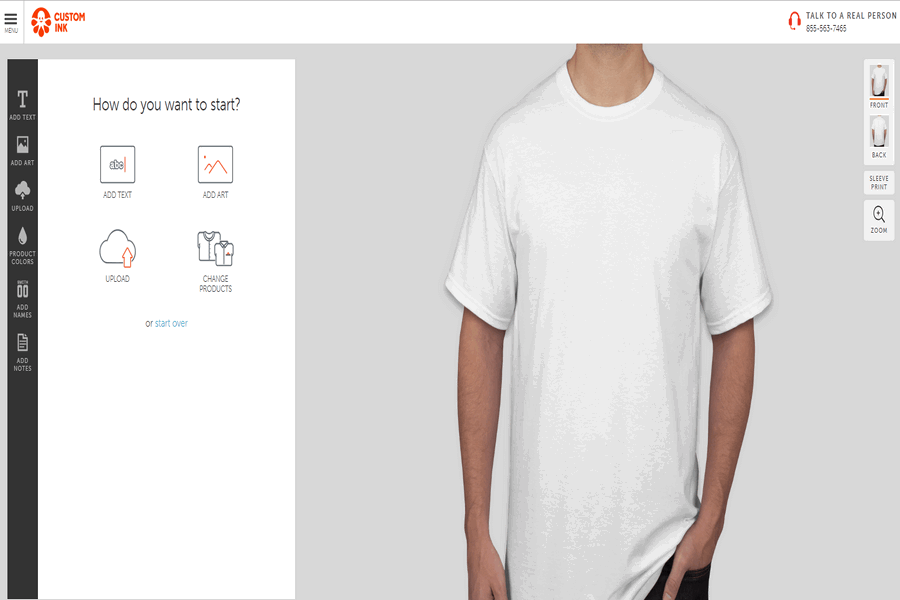The image features a web page from Custom Ink. At the top of the page is a white banner with the text "Custom Ink" written in orange, accompanied by a circular logo. To the left of the banner, there is a menu, and to the right, a message in gray reading "Talk to a real person" with an orange headset icon and the phone number 855-563-7455.

In the main section of the web page, there is a large photograph showing an individual in a plain white t-shirt, standing against a gray background. The person's left hand is in their jean pocket with just the thumb visible, and their head is cropped out of the frame, showing only their neck.

On the left side of the photograph, there are options prompting the user on how to start their design: an "Add Text" button, an "Add Art" button, an "Upload" button depicted with a cloud and an upward arrow, a "Change Products" button featuring folded t-shirts, and a "Start Over" blue hyperlink. Additionally, a black panel on the far left of the screen lists options such as "Add Text," "Add Art," "Upload," "Product Colors," "Add Names," and "Add Notes."